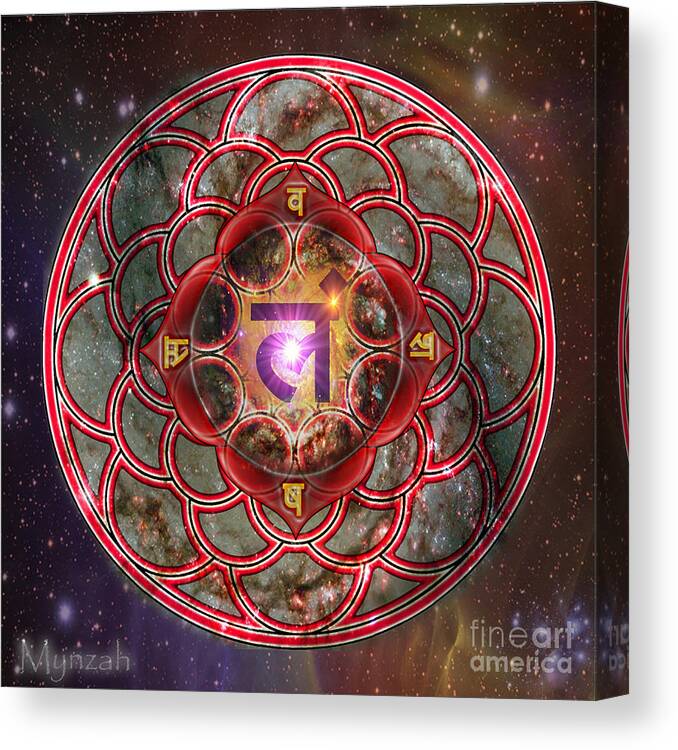This canvas artwork by Fine Art America features the artist's signature "Minza" (M-Y-N-Z-A-H) in the lower left corner. The background is a mesmerizing starry space scene adorned with vibrant nebula-like colors in hues of orange, yellow, and purple. At the center of this cosmic expanse is a prominent circle filled with overlapping and concentric circles that guide the eye to an almost diamond-shaped focal point outlined in red. Radiating from the center, a sun emits beams of purple light that filter through a central symbol, with additional symbols positioned in the cardinal directions—north, east, south, and west. The intricate design of the circles and symbols, characterized by red, white, and black hues, suggest influences reminiscent of Indian or Middle Eastern motifs, lending a rich cultural layer to the piece.